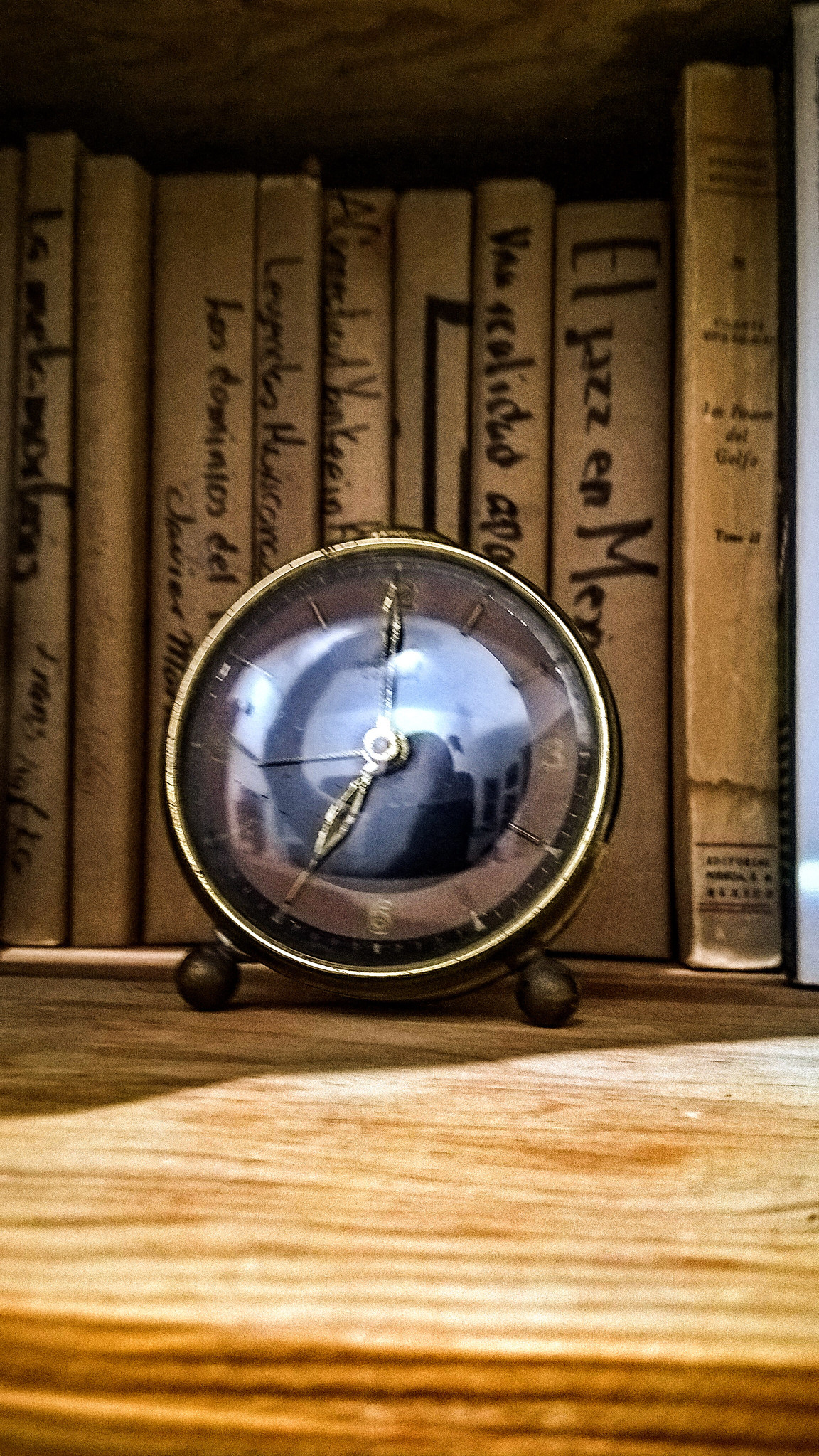Centered on a tan oak bookshelf, the photograph showcases an antique gold analog clock with manual hands, indicating the time at 7 o'clock. The elegant clock features two small, spherical-footed legs, providing stability and adding to its vintage charm. Surrounding the clock are eight to ten books, uniformly covered in a brown wrapper or paper. The spines of these books display handwritten titles in a foreign language, inscribed with a thick black marker, adding an air of mystery and scholarly allure to the scene.